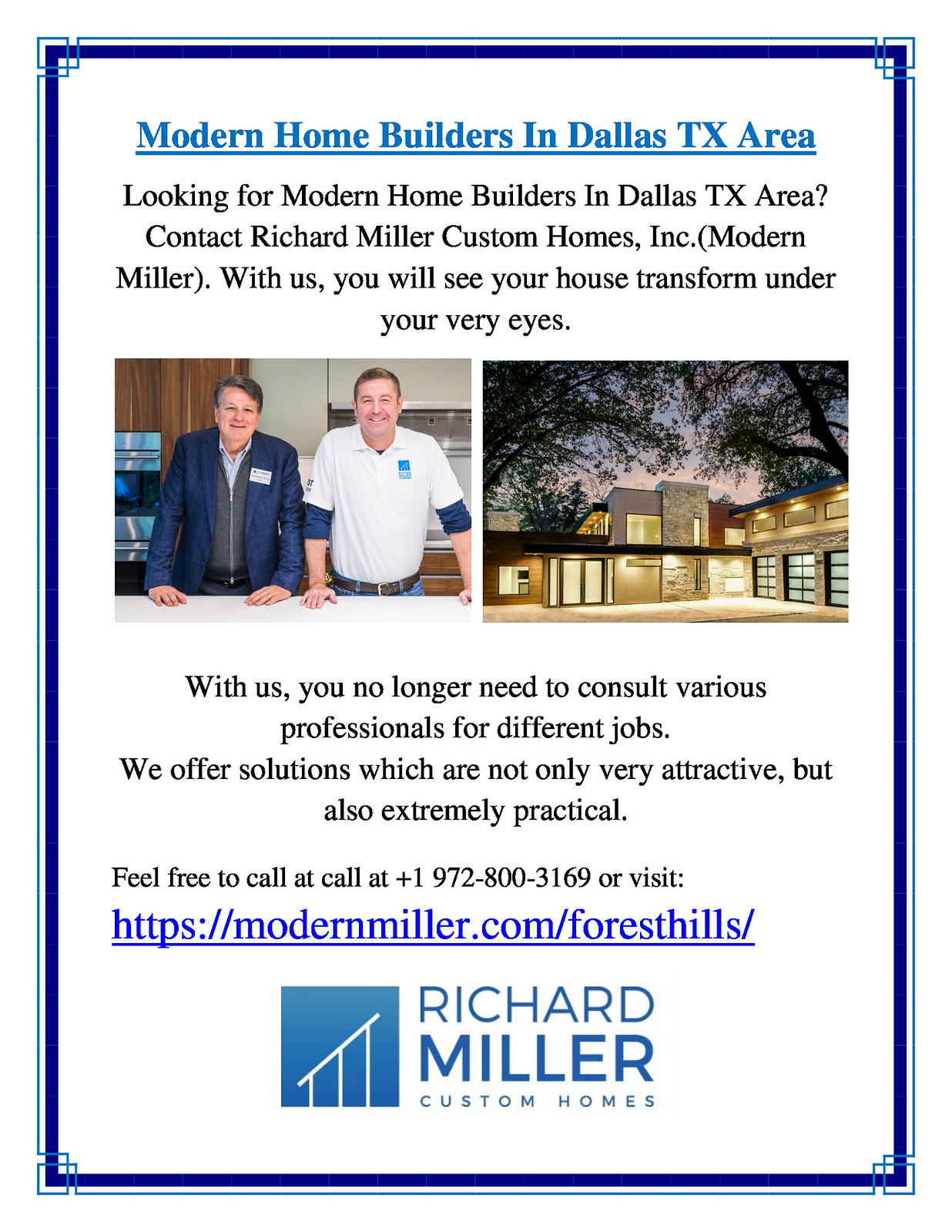The promotional flyer has a white background framed by a blue border. At the top, blue underlined text reads, "Modern Home Builders in Dallas TX Area." Right below, in black text, it states, "Looking for Modern Home Builders in Dallas TX Area? Contact Richard Miller Custom Homes, Inc., Modern Miller. With us, you will see your house transform under your very eyes." The flyer includes two photographs: on the right, a modern, square-like house, and on the left, two people leaning on a counter in a stylish kitchen. Below these images, additional black text highlights, "With us, you no longer need to consult various professionals for different jobs. We offer solutions which are not only very attractive but also extremely practical." At the bottom, contact information is provided in black and blue text: "Feel free to call at 1-972-800-3169 or visit https://modernmiller.com. Forest Hills." The flyer is signed off with a blue logo and the name "Richard Miller Custom Homes."